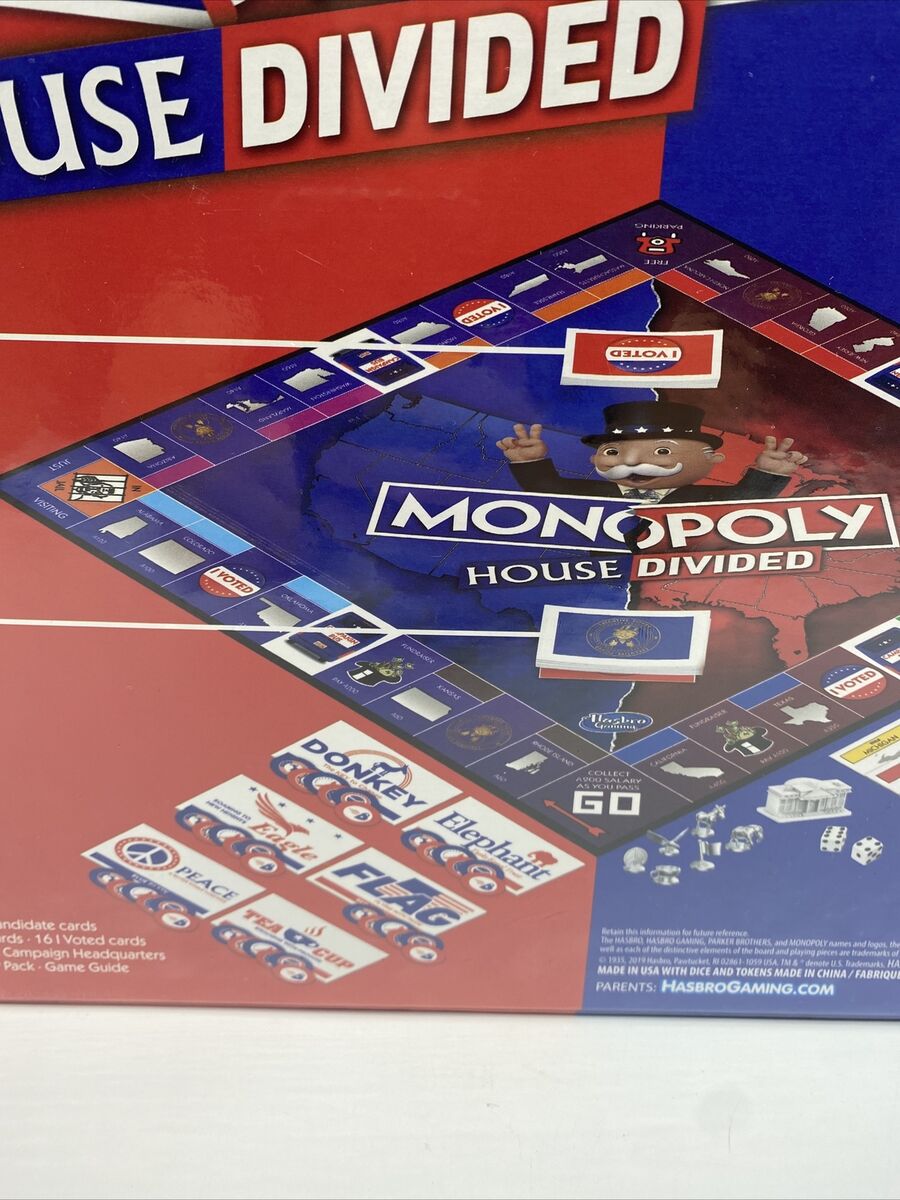The image showcases a Monopoly board game version called "House Divided," which serves as a political satire reflecting the divisions in the United States. The board is bisected diagonally into two distinct color sections: blue on the left and red on the right. The top left of the image features the words "use" and "divided" in white ink, with "use" bordered in blue and "divided" bordered in red.

On the board, you see the typical Monopoly layout, but with states replacing the usual avenues. Classic spaces like "Jail" and "Free Parking" remain, alongside chance and community chest cards with different names. The board displays mascots and tokens fitting the political theme, including a donkey, an elephant, an eagle, a flag, a cup, a White House, and possibly a coin. There are also dice and an "I Voted" sign.

Additionally, the board has the text "Monopoly House Divided" prominently written on it. The image includes information about the game being sold by HasbroGaming.com, noting that it is made in the USA, with dice and tokens manufactured in China. At the bottom right, a dice roll can be seen, and at the bottom left, details about producers or sponsors are visible. Notably, the symbolic figure of the old man in the top hat is depicted with his fingers up in a style reminiscent of Nixon.